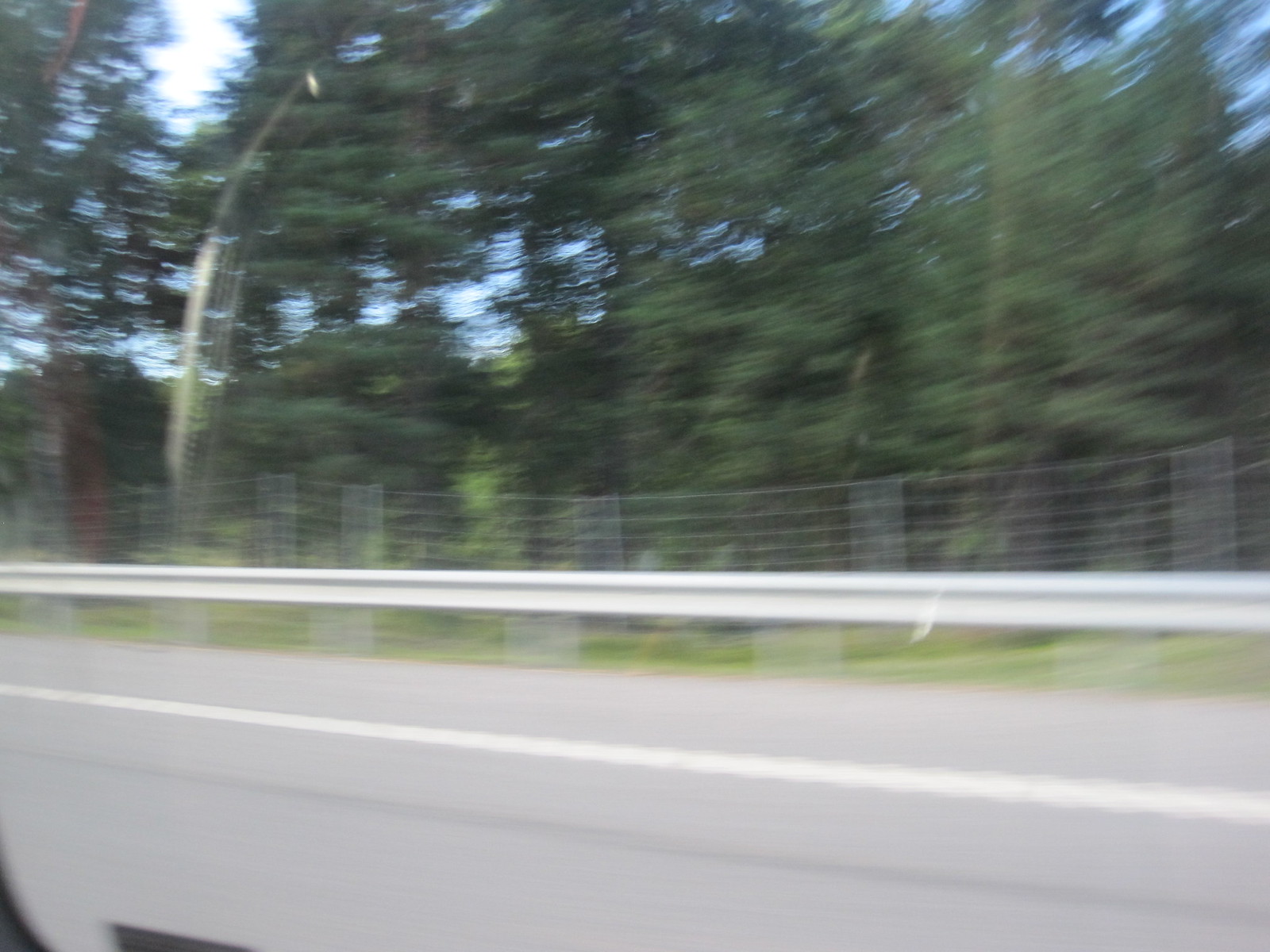This image captures a blurred scene, likely taken from a moving vehicle such as a bus, van, SUV, or car. The photograph's motion blur indicates that the camera's shutter speed was not quick enough to freeze the action. In the bottom left corner, the edge of the vehicle's window is visible along with a faint reflection of the interior, including a hint of red and possibly a woman's head. The primary focus of the image is the landscape outside the vehicle: 

- **Foreground:** The image shows a section of pavement with a white fog line separating the road from the shoulder.
- **Middle Ground:** A metal guardrail supported by vertical posts follows the road's edge, and beyond the guardrail, a mesh fence is visible, potentially for keeping animals off the road or containing livestock.
- **Background:** There is a stretch of grass between the fence and a collection of trees, varying in shades of green with some patches of greenery visible in between. The trees extend into the background, where glimpses of the sky can be seen through the branches and leaves.

This dynamic and detailed scene combines elements of transportation, road safety, and the surrounding natural environment, all depicted with the characteristic blur of motion photography.